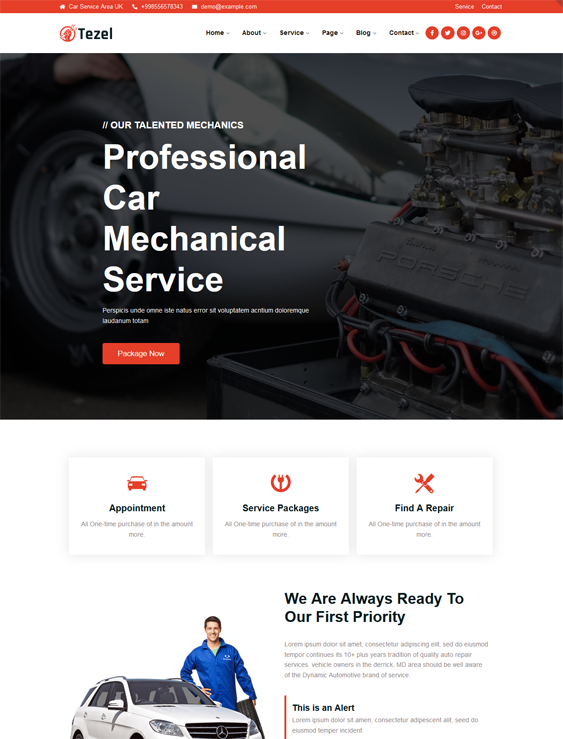In this image, we see a comprehensive layout of a website for a brand named TEZEL. The top section features an orange background divided into three segments on the left side and two on the right. On the far left, the brand's name "TEZEL" is prominently displayed in bold text, accompanied by an orange logo to its left. Below the orange background, there are six categories in black text: Home, About, Services, Pages, Blog, and Contact. Additionally, five social media icons are housed within orange circles on the right side, set against a white backdrop.

The main body of the screen is split into two sections. The upper section showcases a dynamic holographic background with images of a car and an engine, conveying a theme of high-quality automotive care. Centered on this background is the bold text "Professional Car Mechanical Service," accompanied by an orange rectangle at the bottom with the call-to-action "Package Now."

The lower section features three distinct options arranged horizontally from left to right: Appointment, Service Packages, and Find a Repair. At the bottom of this section, a motivational phrase "We are always ready to ... we are always ready. Our first priority" is prominently displayed. Beneath this, two sentences in light gray text provide additional information, though they are quite small and less noticeable.

To the left of the final section, there is an image of a man dressed in a blue jacket standing next to a car, which appears to be a Mercedes SUV, adding a personal touch and a sense of reliability to the website's overall design.